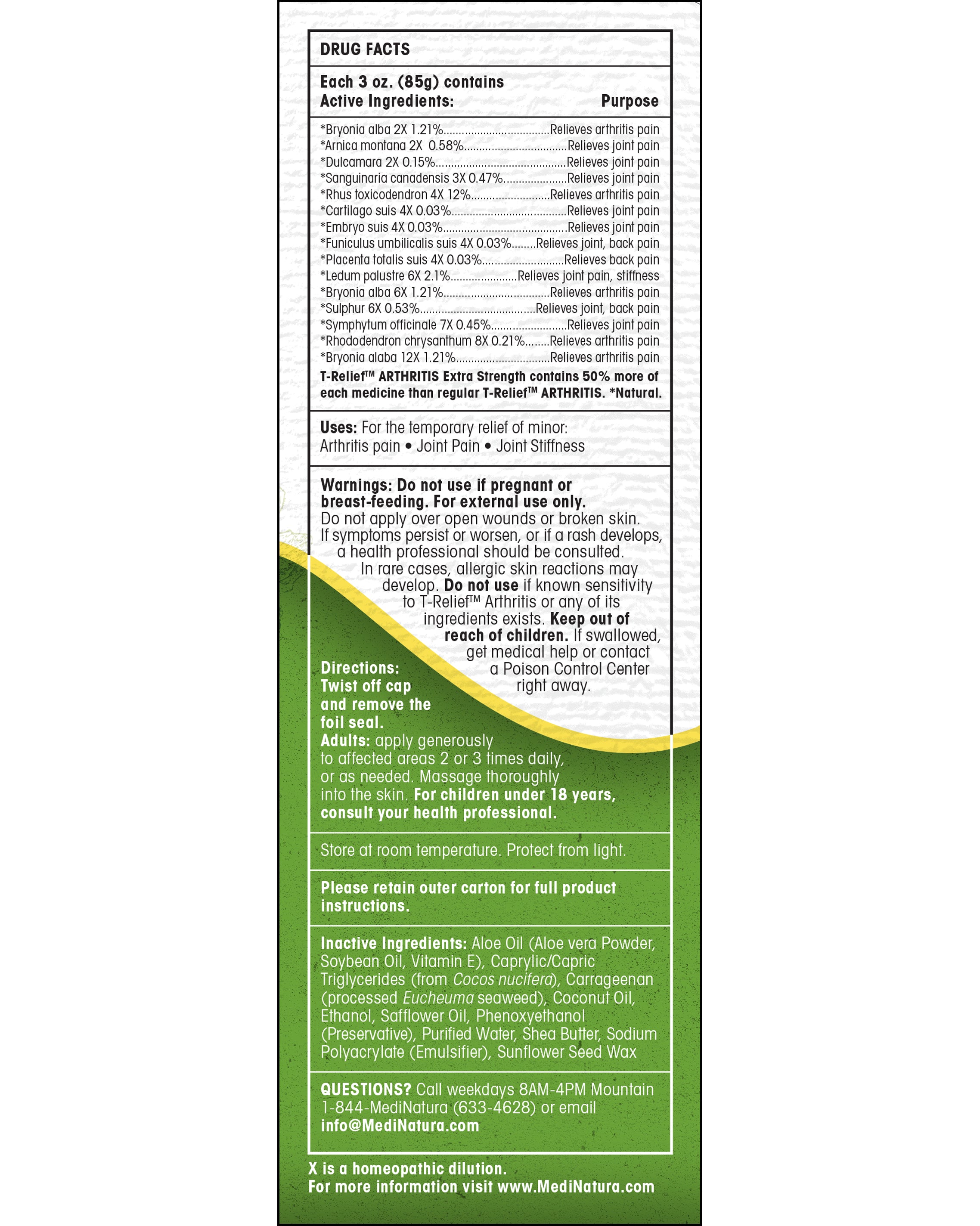The image depicts the back of a box for a joint relief cream or lotion, detailing its drug facts and usage instructions. The top portion of the box, which is white, lists the active ingredients and their purposes for relieving minor arthritis pain, joint pain, and stiffness. This section also includes multiple warnings: do not use if pregnant or breastfeeding, for external use only, do not apply over open wounds, and consult a health professional if symptoms persist or a rash occurs. Users are advised to keep the product out of reach of children and to contact poison control immediately if swallowed. 

A yellow curved line separates the white top from the green bottom section of the box. Below the line, the directions on a green background advise users to twist off the cap, remove the foil seal, and for adults to apply generously to affected areas 2-3 times daily or as needed, thoroughly massaging into the skin. For children under 18 years, consultation with a health professional is necessary. Further guidelines include storing the product at room temperature, protecting it from light, and retaining the outer carton for complete product instructions.

The bottom section also lists the inactive ingredients and provides contact information for further questions, including a phone number, email (info@medinature.com), and operating hours (weekdays from 8 am to 4 pm MT).